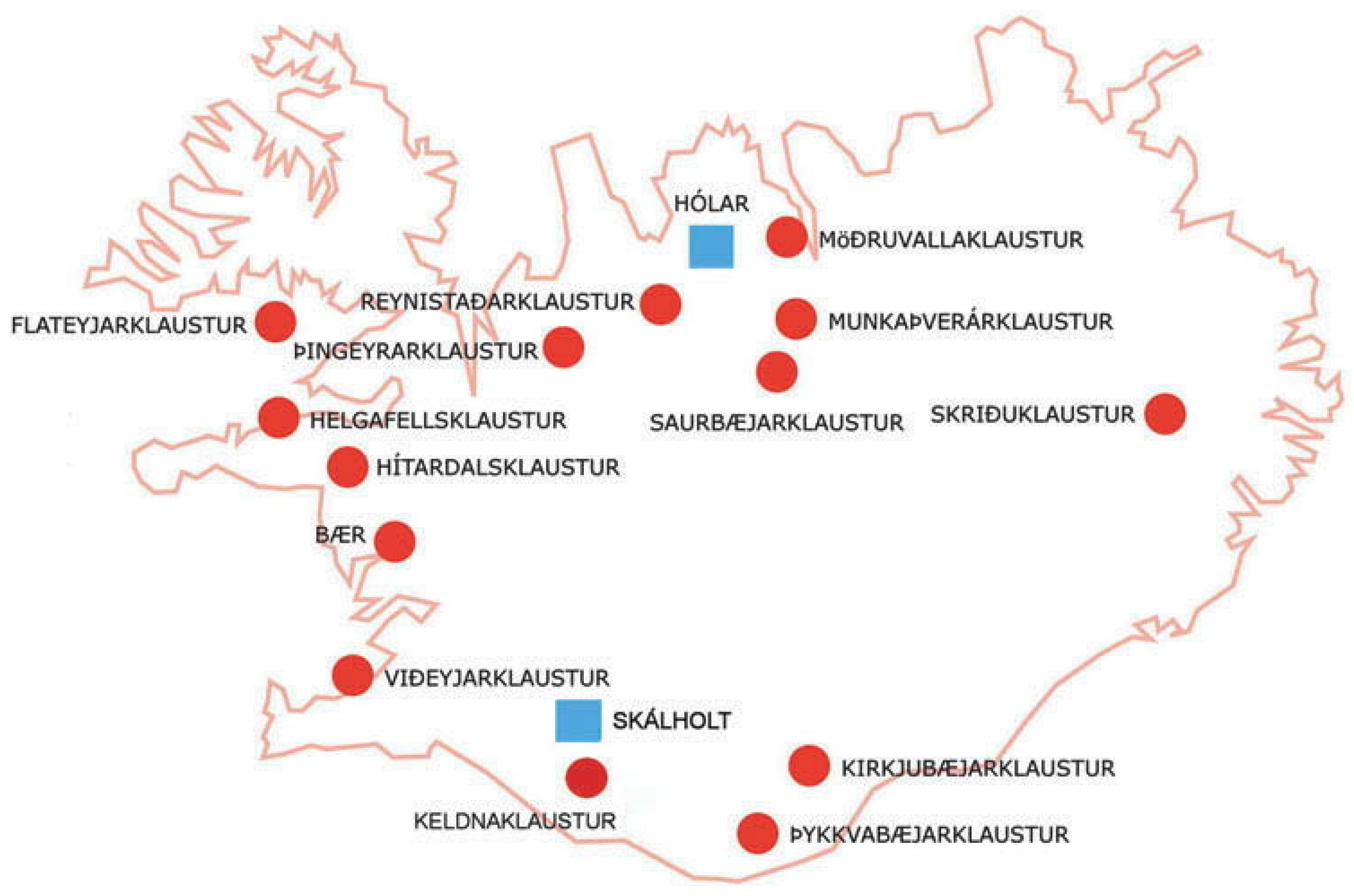This is an intriguing map with white background and a jagged-edged outline, rendered in a light peach or very light brown color, possibly representing a country. Scattered across this map are numerous red dots and two blue squares. Each red dot is accompanied by a name in a foreign language, written in black, which could indicate cities or villages, though the exact country or language is unclear. Notably, the blue squares mark two specific locations named Hólar at the very top and Skálholt at the bottom of the map. The language of the names is unfamiliar, and attempts to identify it suggest it could be Swedish, Finnish, or potentially something entirely different, perhaps even fictional.